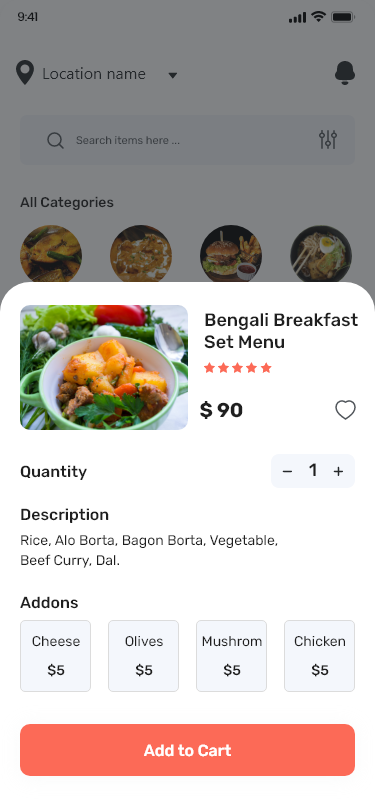Screenshot Description:

The mobile app screenshot displays the detailed view of a menu item that is currently selected. At the bottom of the screen, there is a highlighted section featuring the "Bengali Breakfast Set Menu." To the left of this menu title, there is an appetizing image of a meal, which includes what appears to be potatoes, spinach, tomatoes, carrots, and pieces of meat.

The price of the Bengali Breakfast Set Menu is listed as $90. Above the price, the meal boasts a perfect rating of five out of five stars, indicated by five vibrant orange stars. To the right of the rating, there's a heart icon, presumably for users to like or love the dish. Below the menu title, there is an option to adjust the quantity, displayed as "1" by default, with a minus and plus sign on the left and right sides respectively to decrease or increase the quantity.

The description of the meal is comprehensive, listing the main components as rice, alo borta, bagan borta, vegetable, beef curry, and dal. The optional add-ons are listed below, each priced at $5: cheese, olives, mushrooms, and chicken. An oblong, orange-red button with white font is situated below the description, featuring the text "Add to Cart," making it easy for users to add the item to their shopping cart.

Behind the clipped part of the screenshot, the top part of the app features a location name with a dropdown menu for selection. To the right of it, there's a notification bell icon. Below these elements, there is a search bar with a magnifying glass icon on the left side and a settings button on the right. Further down, the app displays "All Categories" with four images of different food types. One image clearly shows a burger, another depicts ramen with chopsticks, while the other two images are somewhat obscured and grayed out, making it difficult to identify their contents.